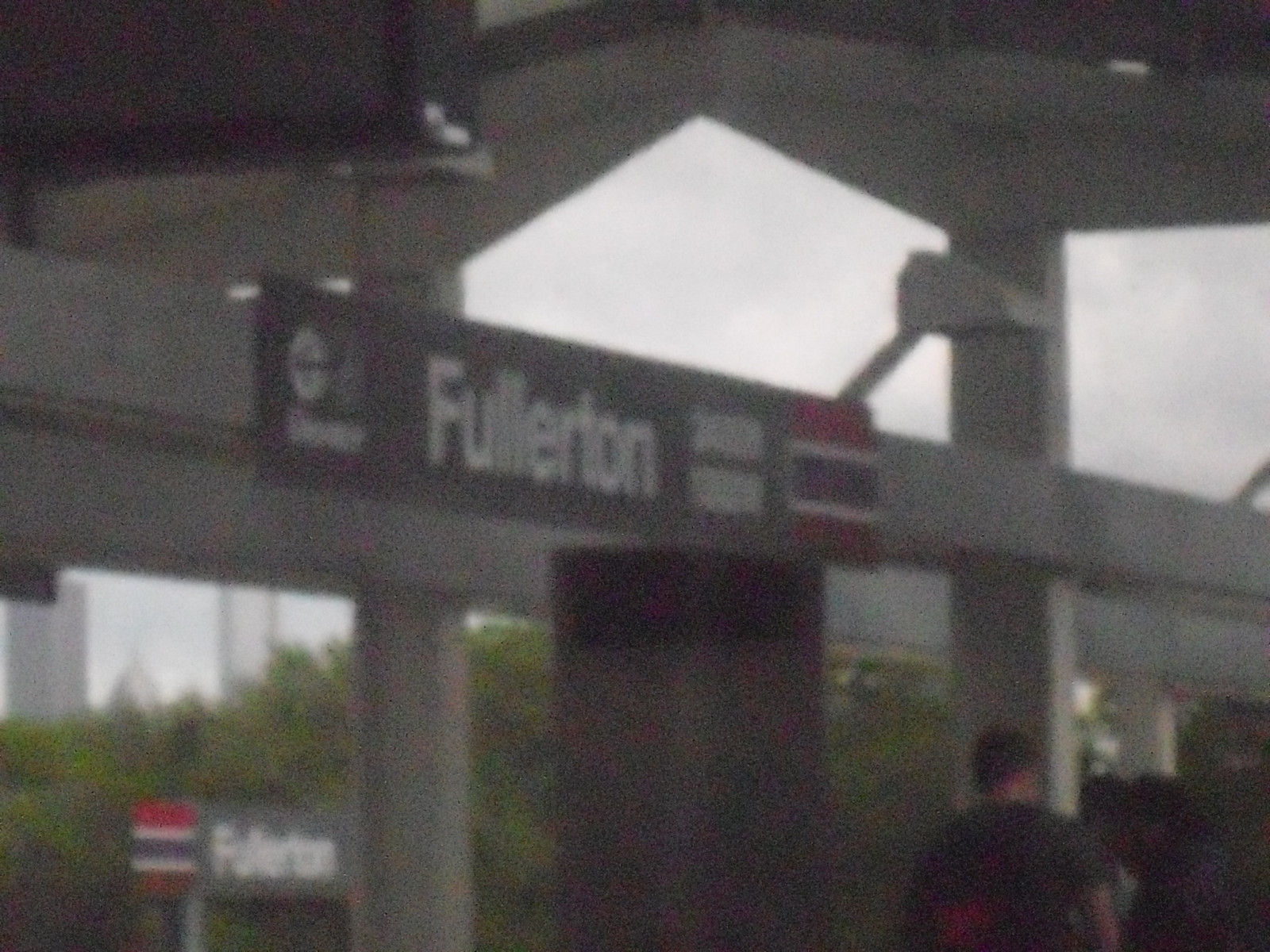Under a large, open canopy, this grainy, slightly out-of-focus image captures a scene featuring concrete pilings horizontally arrayed above. In the middle of the image, a rectangular sign with white text boldly announces "Fullerton." Below and to the right, another sign, likely resting on the ground, also bears the name "Fullerton." The background is tinged with green, hinting at the presence of bushes or trees, adding a touch of nature to the otherwise industrial scene. In the bottom right corner, the vague silhouettes of two or possibly three people can be discerned, their forms and coloring barely distinguishable due to the image's quality. Above, a light gray sky stretches across, completing the ambient setting of this outdoor location.